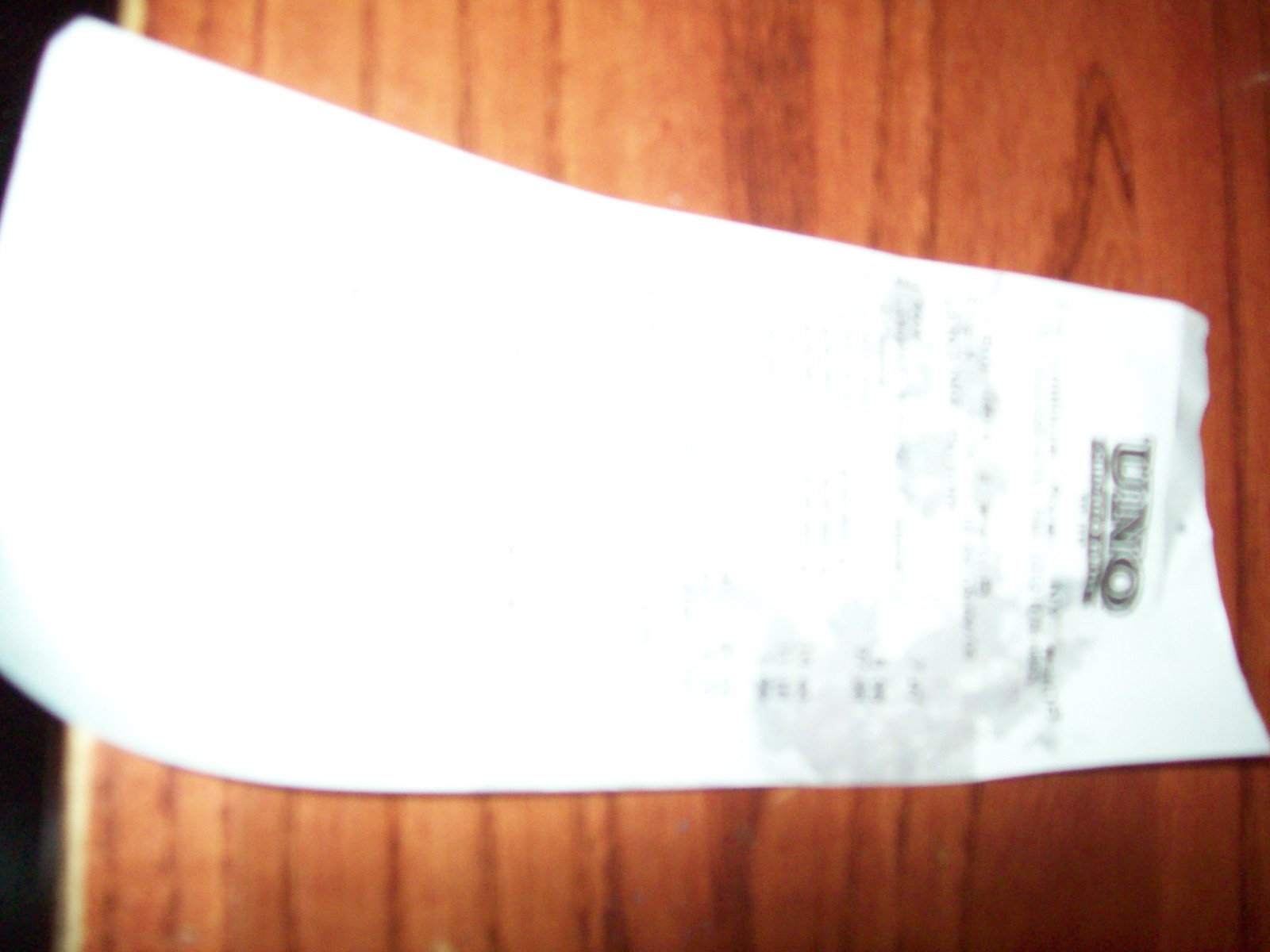A blurred, rectangular image displays a receipt laying on a medium-brown wooden tabletop, oriented horizontally with the long side extending from left to right. The receipt itself runs from right to left within the image. The text at the top of the receipt, despite the blur, appears to spell "UNO" in black letters, with the rest of the receipt's content also printed in black on a white background. The distinctive wood grain of the tabletop is visible, adding texture to the scene. On the left edge of the photo, a dark black area stands in contrast to the rest of the composition.